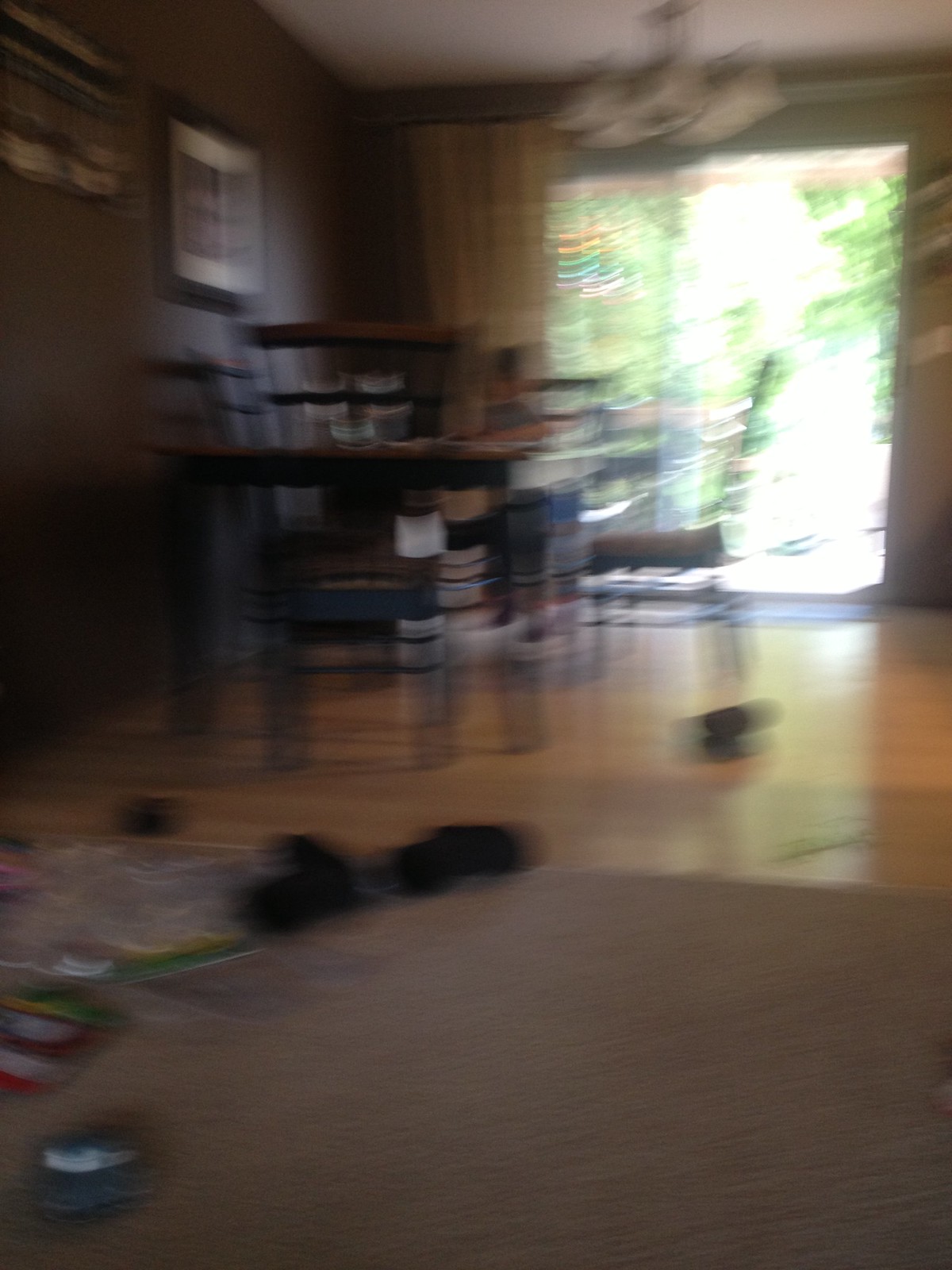This photograph, albeit blurry, captures the inside of a cozy home, viewed from a living room peering into the kitchen area. In the foreground, a wooden floor is partially visible, scattered with various items such as shoes and socks, hinting at a lived-in, family-oriented space. A carpet area near the bottom of the photo is cluttered with additional items, potentially toys, adding to the homely disarray.

At the center of the image, a kitchen table surrounded by chairs stands on the wooden floor, signifying the heart of the home where meals and moments are shared. In the background, a sliding glass door, bathed in sunlight, offers a glimpse into the verdant outdoors. Green trees flourish in the bright daylight, signaling a vibrant, sunny day. Hanging outside on the back porch, a colorful wind chime or similar ornament sways gently, adding a touch of whimsy to the serene scene. Despite the blurriness, the photograph exudes warmth and the essence of daily life within a welcoming home.